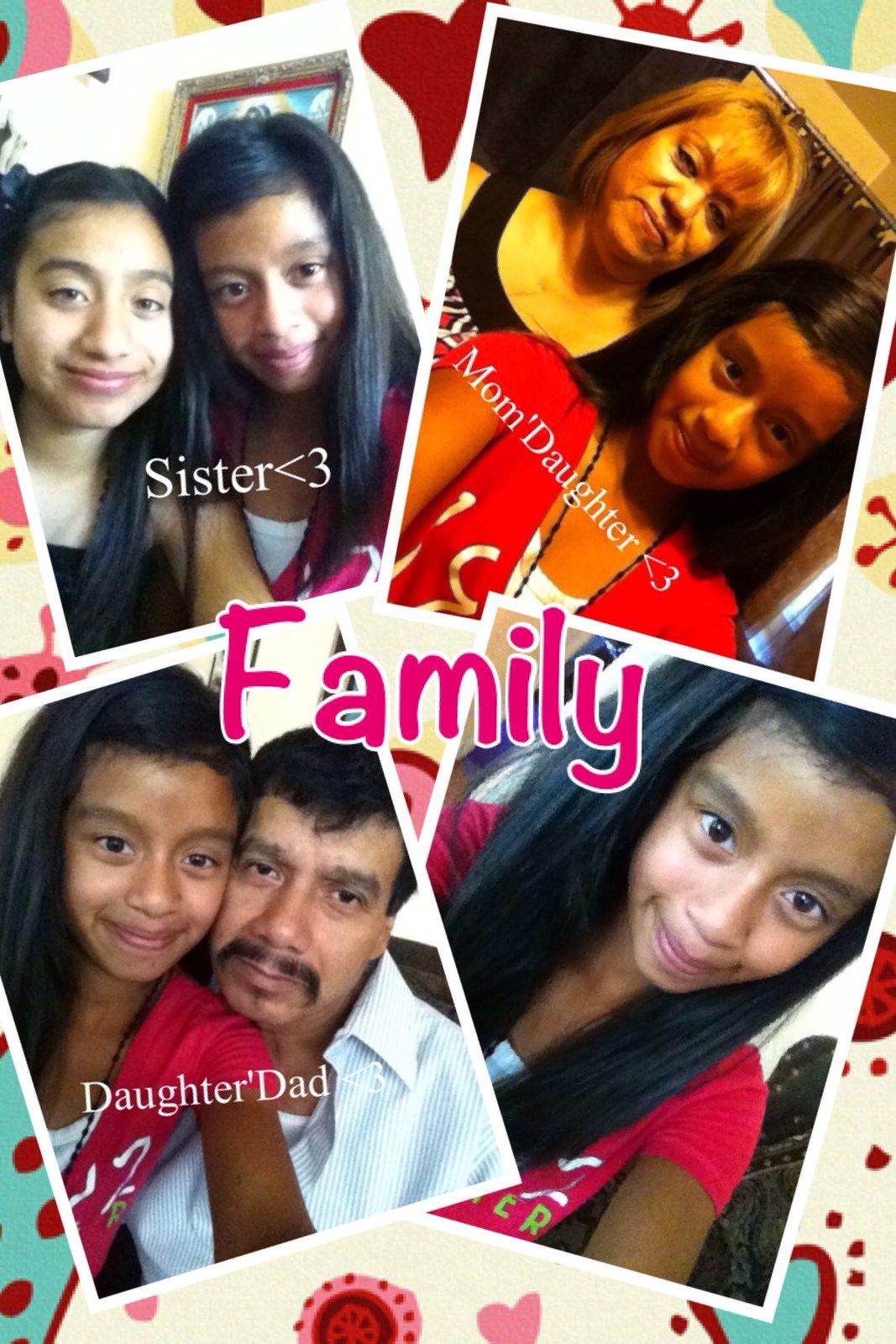This image features a thoughtfully composed collage of four family portraits, arranged diagonally with a slight tilt, creating a dynamic yet organized layout. Centered prominently within the collage is a large, pink "Family" text. The four photos are framed with white borders and are set against a whimsical background of colorful heart designs.

- The top left photo showcases two sisters with long, dark hair, smiling warmly with their heads close together.
- The top right photo captures a tender moment between a mother, bathed in a yellowish tint, and her daughter.
- The bottom left photo depicts the daughter with her father, who has short black hair and a mustache, both looking directly at the camera.
- Finally, the bottom right photo features the daughter alone, highlighting her straight black hair and red clothing, which she wears in all the pictures.

The backdrop of the collage adds a playful touch with various illustrations and graphic elements, enriching the overall family theme. The intricate details and harmonious color scheme emphasize the close-knit bond shared by the family members.